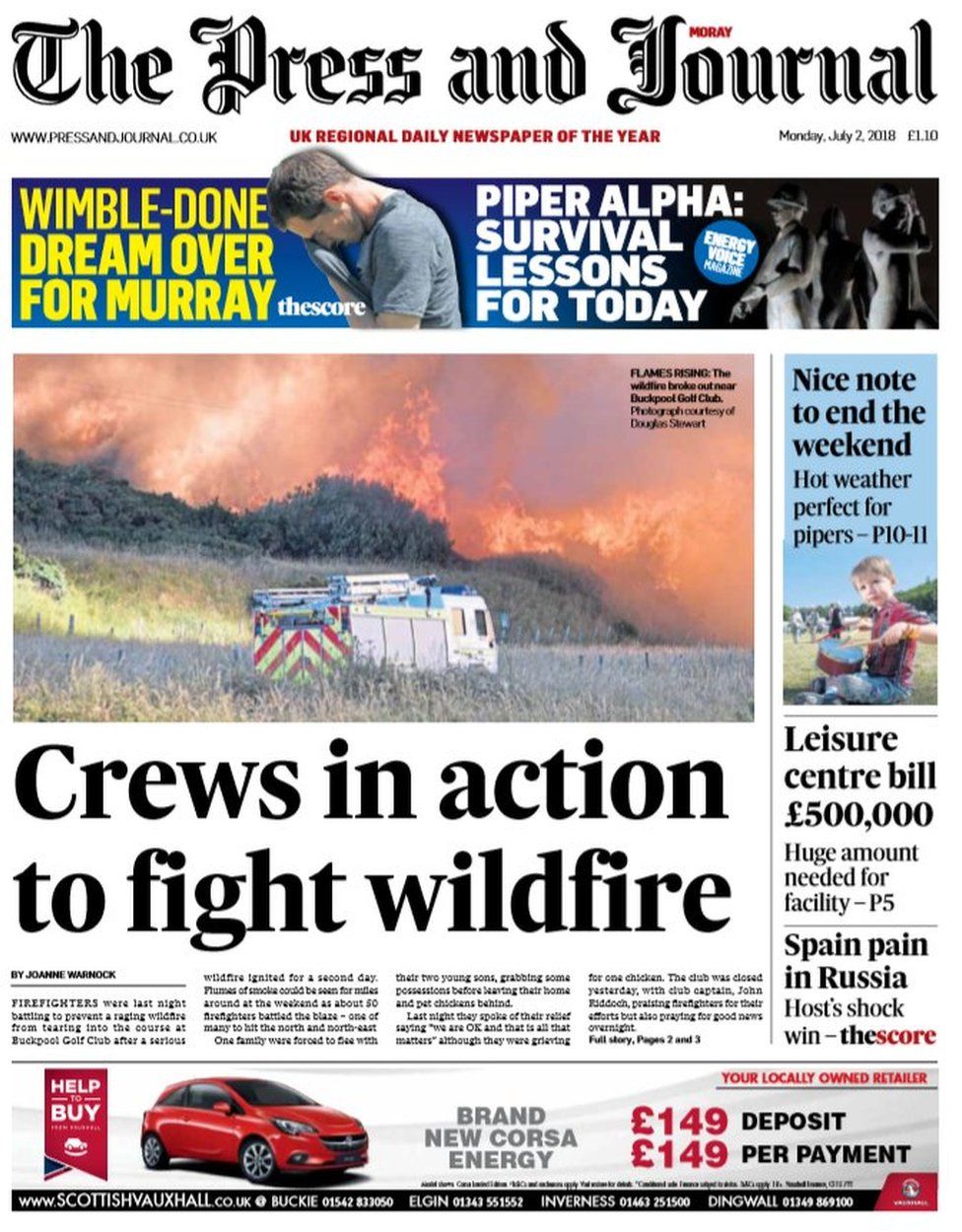**Front Page of the Press and Journal - Monday, July 2nd, 2018**

At the top of the page, the newspaper's title, "Press and Journal," is elegantly presented in an ornate black font, with "M-O-R-A-Y" written above in red letters. Below the title line, additional information is displayed: the website address "www.pressandjournal.com.uk," accolades including "UK Regional Daily Newspaper of the Year," the date "Monday, July 2nd, 2018," and the price "1 pound 10 pence."

**Main Image and Headline**
The central focus of the front page is an intense photograph of a wildfire. Flames and thick smoke rise dramatically from a hilly area, partially obscured by vegetation. An emergency vehicle is stationed prominently in the foreground, highlighting the urgency of the situation. The headline, "Flames Rising," is positioned at the top right of the photo. The wildfire reportedly erupted near Duck Pool Golf Club, with the photograph credited to Douglas Stewart. A subheadline reads, "Crews in Action to Fight Wildfire."

**Additional Feature Stories**
To the left of the main image, yellow letters headline "Wimble Done, Dream Over for Murray," accompanying an image of a distressed white man. He appears to be wiping his face with his gray short-sleeved shirt, his head bent in apparent defeat.

To the right, a black and white image depicts a statue of soldiers, with the headline "Piper Alpha, Survival Lessons for Today."

**Inset Photographs and Stories**
In the top right corner, a small photograph captures a little boy on a grassy patch, energetically playing a drum with drumsticks. The caption beneath reads, "Nice Note to End the Weekend, Hot Weather Perfect for Pipers," and directs readers to pages 10-11 for more details.

Further down, a headline addresses financial concerns: "Leisure Center Bill, 500,000 pounds, Huge Amount Needed for Facility," which can be found on page 5.

Another sporty update is headlined "Spain Pain in Russia, Host's Shock Win," briefly summarizing a significant match outcome.

**Advertisement**
At the bottom of the page, a bold advertisement features a two-door red car parked at a slight diagonal, its front end facing right. The ad promotes a "Brand New Corsa Energy" from a locally owned retailer, offering a payment plan of a "149-pound deposit" and "149 pounds per payment." Contact details and website information are provided: "www.scottishvohaul.com.uk" along with phone numbers for locations in Buckie, Elgin, Inverness, and Dingwall.

This detailed layout offers a comprehensive glimpse into the notable stories and visual elements featured on the front page of the Press and Journal for July 2, 2018.